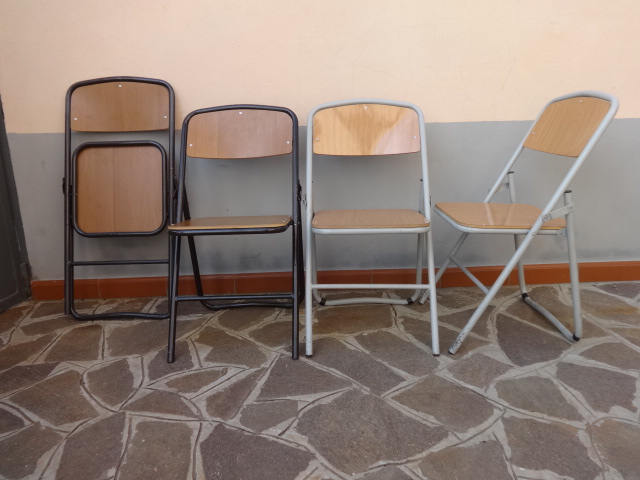The detailed photograph captures an indoor hallway featuring a patterned carpet that mimics tile. This hallway displays a wall with a two-tone color scheme: the upper portion is painted peach, while the lower portion is gray and runs along wood molding at the base. Arranged against this wall are four folding chairs, their arrangement and design sets providing distinct visual interest. 

On the left side, the first chair is fully folded and leaned against the wall, featuring a black metal frame with a wood or engineered wood seat and backrest. The second chair, identical in design, is fully open and positioned next to it. The right side hosts two additional chairs, each with a gray metal frame and a similar wooden seating structure. Both are open and ready for use. The gray-framed chairs are positioned very close to each other against the pale-colored wall that transitions to gray at the bottom.

The floor’s patterned carpet contrasts subtly with the brown and gray of the chairs and walls, adding texture and interest. The setup potentially suggests a small meeting room or waiting area, underscored by the neat arrangement of the chairs and the clean, orderly space.